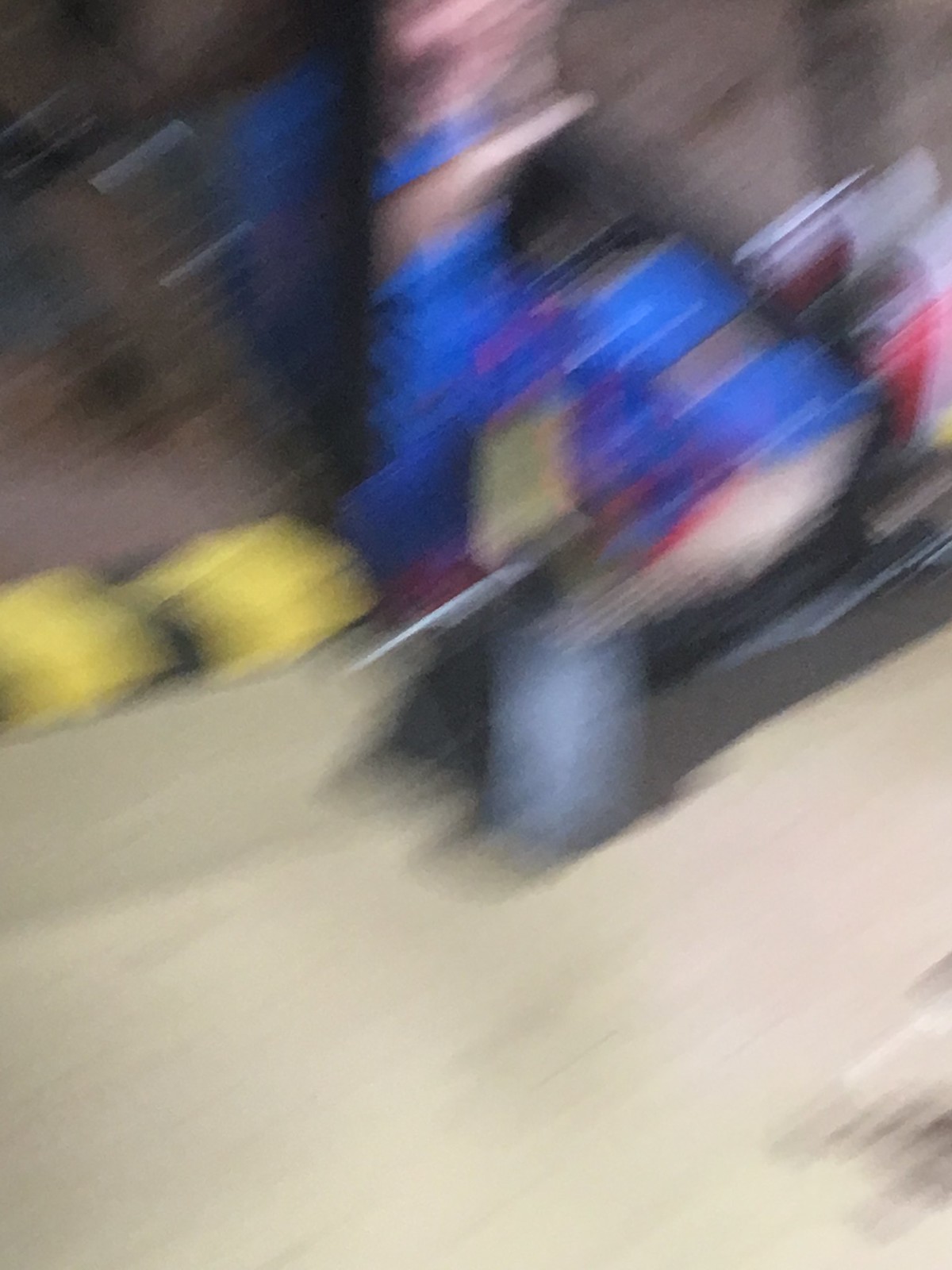The image is extremely blurry, likely caused by fast motion, resulting in a slanted and distorted view. The ground appears beige, occupying the bottom half of the picture. Above that, there are two distinct yellow shapes, possibly food items or objects, within a beige container. In the center towards the right, there's a shape that is predominantly blue with some peachy skin tone and black areas, giving the impression of a person skiing or sliding down a hill. Additionally, a reddish trim and maroon and white elements are visible, which could resemble shoes. The background is a blurred light brown color. Overall, the image depicts rapid movement with indistinguishable details, but the prominent colors and vague shapes hint at a dynamic scene with possible outdoor or recreational activity.